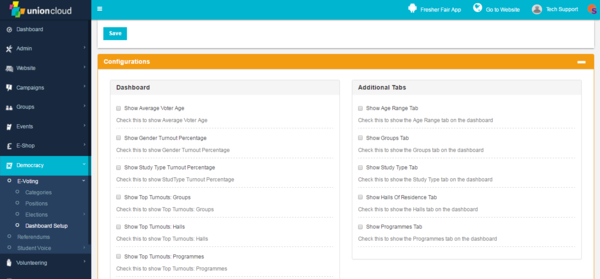In the image, the left-hand sidebar prominently features a menu with multiple items listed in the following order: Union Cloud, Dashboard, Admin, Website, Campaigns, Groups, then CSHOP, Democracy, Unit, Categories, Position, Selection, and Dashboard Setup. At the very top of the interface, a blue bar includes options such as Website and Tech Support. Below this, a series of orange tabs offer various functionalities including Configurations, Dashboard, Show Average Voter Age, Check Digital Average Voter Age, Show Gender Turnout Percentage, Show Study Type Percentage, Show Top 10s of Groups, Show Additional Types, Show Age Range, Show Groups Types, and Show Study Type Types. The background of the interface is predominantly white, with blue highlights corresponding to different column headers. The design is clean and organized, providing a navigable layout for users.